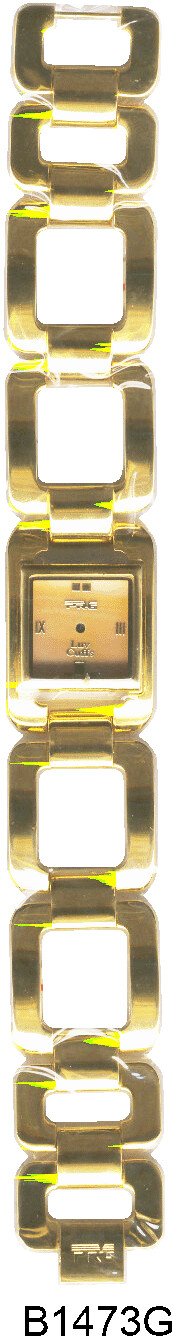This image features a watch with a small face and a sophisticated design. The watch face has a white background with a white gold-tone finish. Roman numerals are positioned at the three o'clock and nine o'clock markers. There are no visible hands on the watch. Intricate writing, which is not legible, is present inside the watch face. Two dark-colored dots mark the 12 o'clock position. The watch's bracelet consists of gold, square-shaped chain links connected by small hinges. The entire object is showcased against a plain white background. In bold black characters at the bottom, the code "B1473G" is displayed prominently.